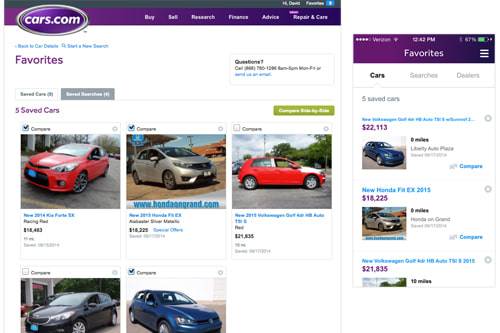The image consists of two sections, both set against white backgrounds. 

### Left Section:
At the top, there is a purple header displaying the text "cars.com." Beneath the header are several navigation headings. One of the headings labeled "Favorites" shows three saved cars. They are displayed in a vertical arrangement:

1. A small red car.
2. A gray car.
3. Another small red car.

Below these three cars, there are two additional cars: a black car and a blue car.

### Right Section:
The right section also features a white background with a purple box at the top, indicating the time as "10:42 AM" and labeled "Favorites." In this section:

1. A blue car priced at $22,113.
2. A silver car priced at $19,225.
3. The third car is partially cut off in the image but is still visible.

Each car listing has an associated blue "Compare" button next to it. Additionally, there is detailed information and a picture of each car. Users can click on any of these cars to see more details.